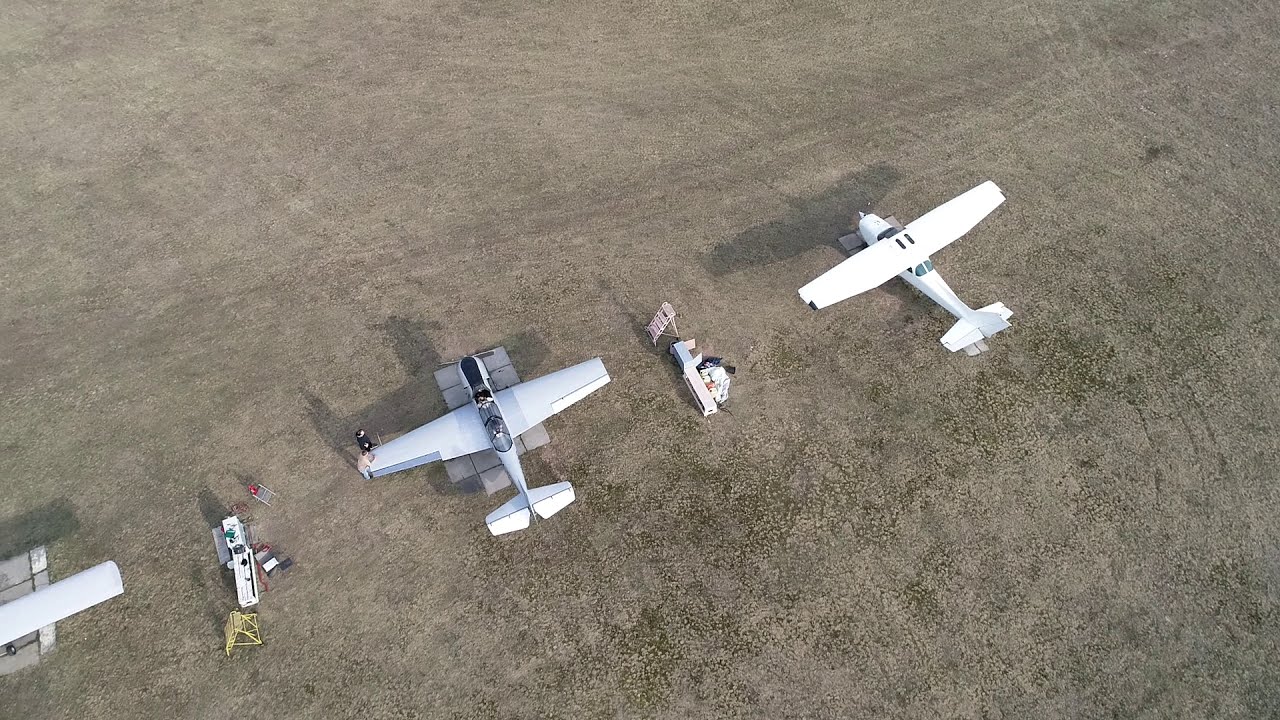This horizontal, aerial photograph captures a small airfield with tie-downs for small hobby planes. Dominating the foreground are two modest white airplanes, flanked on the left by what appears to be a corner of a white hangar building. Between the planes, several white maintenance vehicles and a white stand are visible. A yellow step ladder is positioned next to the left wing of the leftmost airplane, where two people are leaning over, possibly conducting pre-flight checks. In the distance, a red and white bulletin board stands, though it is too far away to make out any details. The background is largely a flat expanse of brown dirt, lightly interspersed with some bushes and patches of green moss, creating a mixed yet predominantly earthy terrain.